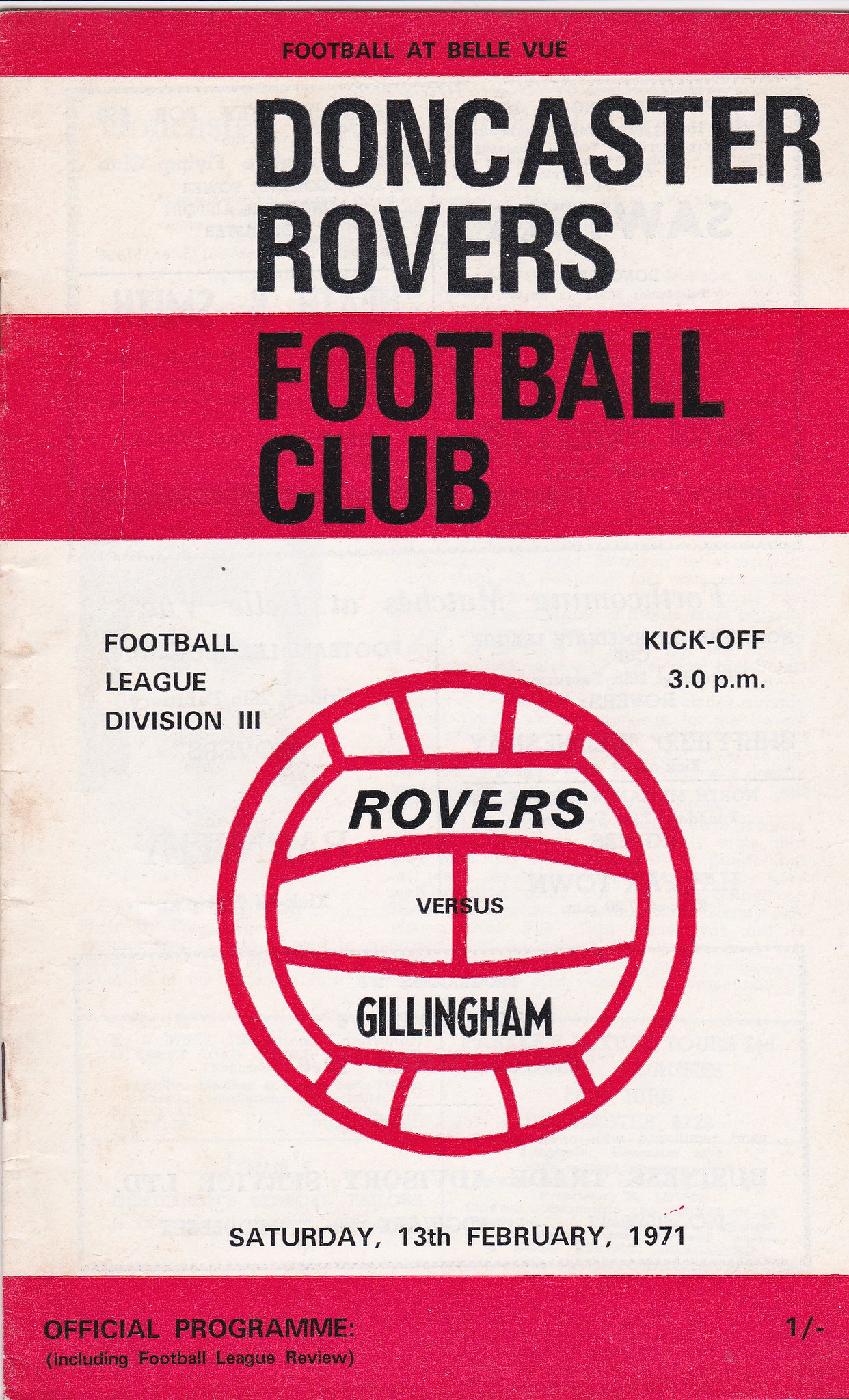This image features the front cover of an official program for a football match. Dominated by shades of red, white, black, gray, and pink, the program prominently showcases its text in black. At the very top, it reads "Football at Bellevue," followed by "Doncaster Rovers Football Club." Centered below this, left-aligned, is "Football League Division 3" with kickoff time indicated as "3 p.m." In the middle of the cover, there are two large white stripes across a red background, emphasizing a soccer ball outlined in red. Centered on the ball is the text "Rovers versus Gillingham." Below this, in black text, is "Saturday 13th February 1971," marking the date of the match. The bottom of the cover notes that this is an "Official Program including Football League Review." This visually nostalgic cover evokes the style of an early 70s football game program.